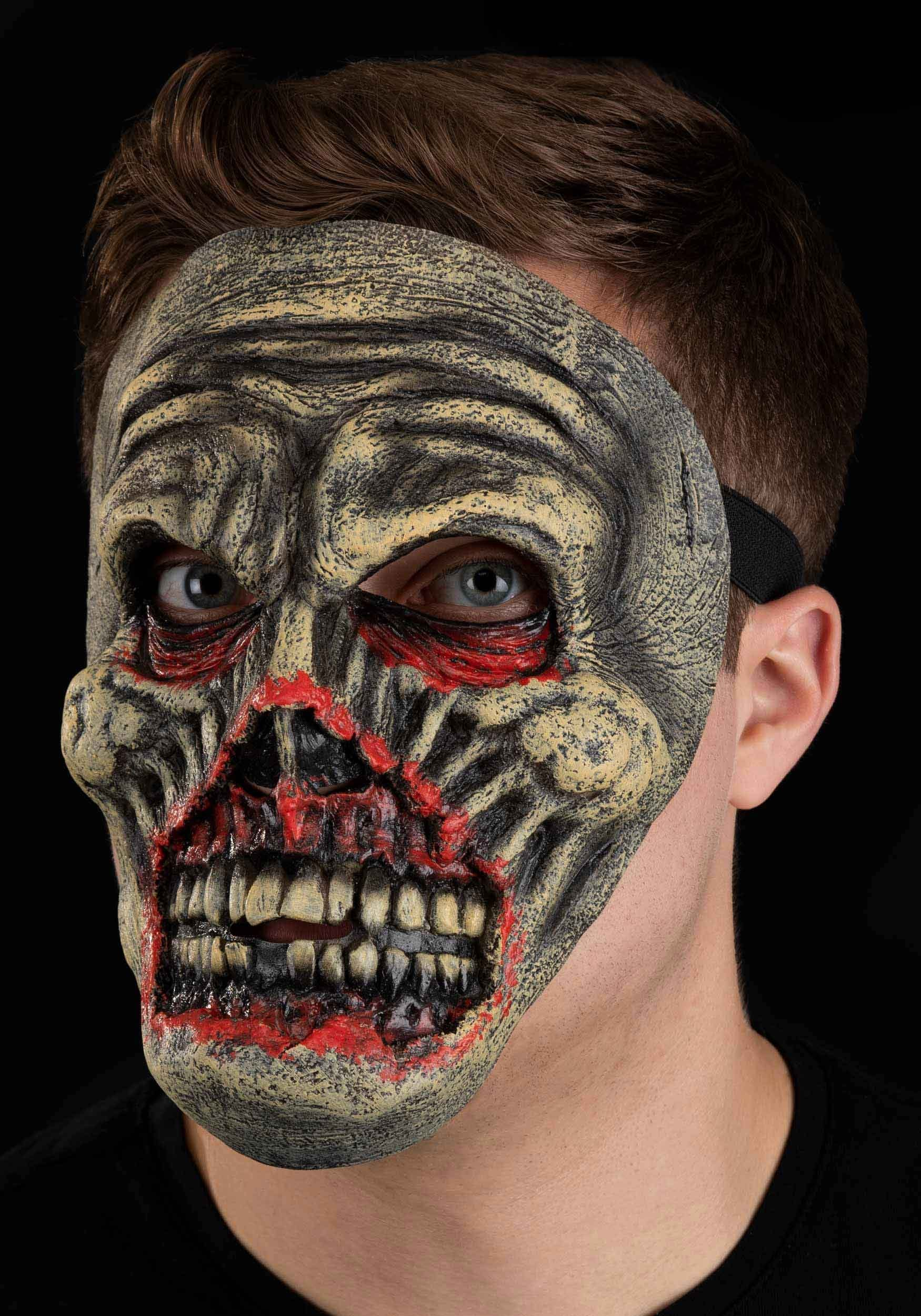The image depicts a man facing the camera, wearing an intricately detailed, weathered skeleton mask that combines elements of a reaper and a zombie. The mask features sunken in bones, exposed teeth, and hollowed eye sockets, with a color palette of black, yellow, red, and gray which gives it a decrepit, eerie appearance. The mask appears gruesome with torn flesh details, shredded areas around the mouth and nose, showing the teeth and nose's interior structure, giving it a grotesque and terrifying look. The man has brown hair neatly trimmed, blue eyes visible through the mask's eye holes, no facial hair, and wears a black t-shirt that blends seamlessly with the dark black background. The mask is secured by a black strap visible on the right side of the image, adding to the overall menacing and detailed appearance of the scene.